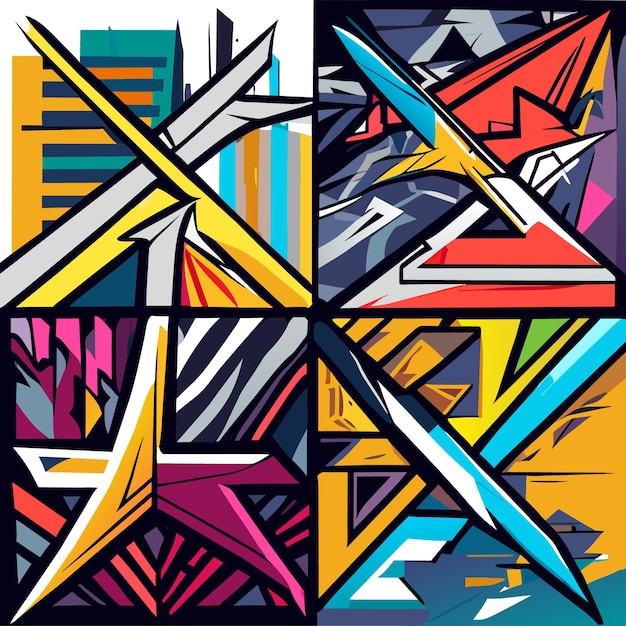This image is divided into four equal sections, each showcasing vibrant, abstract patterns with crisscross shapes and varied color palettes. The top left section features a background of yellow, grayish white, teal, dark blue, light blue, and orange, with horizontal and vertical stripes intersecting to form an X or diamond shape in the center. The top right section displays a mix of red, dark blue, light blue, gray, yellow, and white, arranged in stripes and streaks that also converge into a crisscross pattern. The bottom left section has shapes that resemble a star with dark yellow, white, magenta, navy blue, purple, and pink hues. The lower right section includes light blue, dark navy blue, white, yellow, green, and dark yellow, with the lines and shapes forming an X-like pattern. Each quadrant maintains a unique yet harmonious abstract design, creating a visually striking collage.